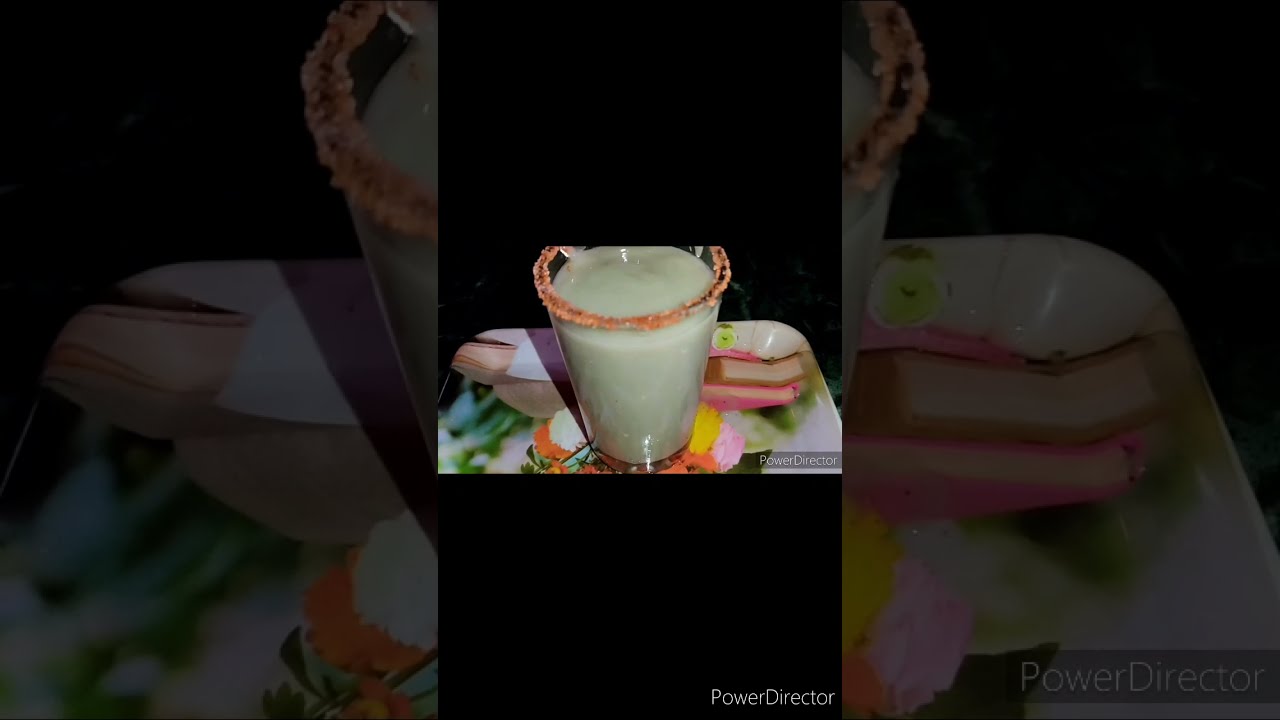The image consists of three panels, with the central one featuring a clear drinking glass on a colorful, flower-decorated ceramic plate. The liquid inside the glass appears greenish-white and has a rim coated with what seems to be colored sugar or a seasoning like Tajin. The top and bottom sections of the central panel are black, framing the image. The side panels are underexposed blow-ups of the central photo and serve as a darkened backdrop. At the bottom right-hand corner, thin white text reads "Power Director."